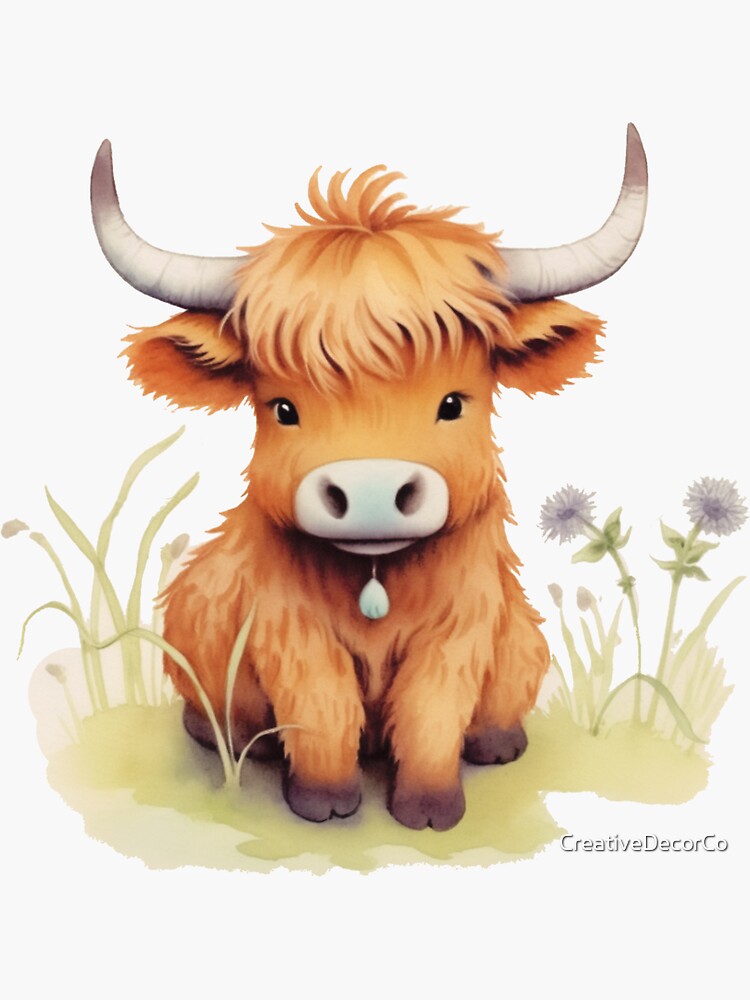The image features a whimsical watercolor painting of a young, brown Highland cow with a shaggy, blonde mane. The cow, characterized by its innocent, wide-set black eyes and half-smile, sits on its hind legs facing the viewer. The cow’s flat ears, also covered in shaggy hair, hang down on each side of its face, which is adorned with a wide nose and pronounced nostrils. Two light gray horns curl upward from its head, with darker gray tips aimed skyward. It wears a collar with a dangling silver pendant. Its front legs, with black hooves that have a distinctive V-notch, are visible. The cow sits on a light green patch of grass, accented with tall blades and a few blue-gray flowers. The backdrop is a light gray, and in the lower right corner, a watermark reads, "Creative Decor Co."